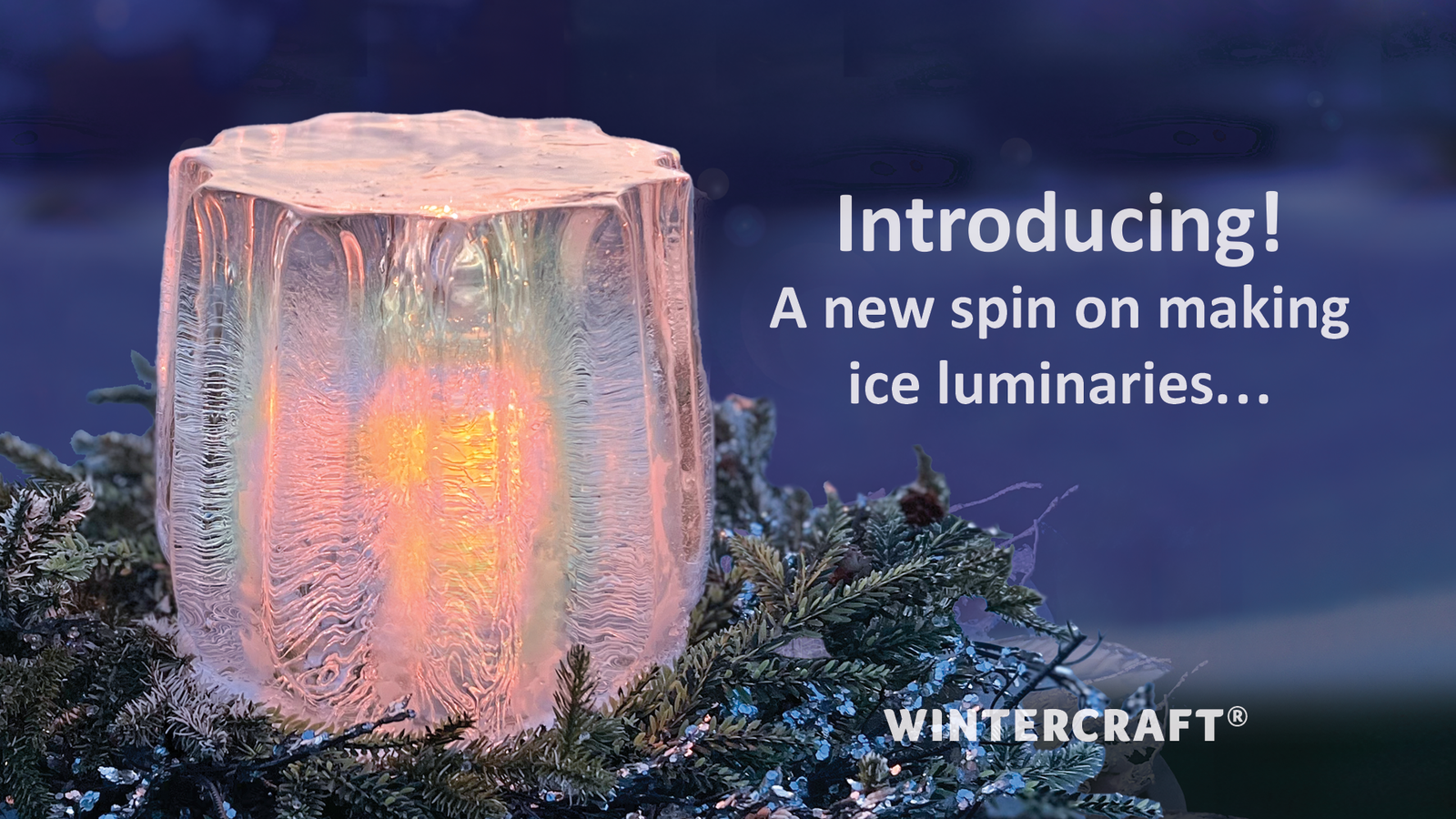This advertisement features a horizontally oriented image with a blurred dark blue background, creating a serene and cool atmosphere. In the foreground, to the left, there is a striking clear glass sculpture resembling an ice luminary. The structure is rounded and about three inches tall, with intricate beveled and fluted edges, giving it a unique texture and shape. The glass has tiny horizontal lines across its surface, obscuring the view inside but allowing a captivating inner glow to shine through. The glow emanates different shades of pink with a touch of yellow at the center, creating a warm, inviting light.

This luminous object is nestled atop a bed of green pine needles dusted with a hint of snow, adding a natural, wintry touch to the scene. The arrangement of the pine needles encircles the glowing luminary, enhancing its visual appeal.

To the right of the image, bold white text announces, "Introducing!" beneath which it declares, "A new spin on making ice luminaries." Below this text, "Wintercraft®" is prominently displayed, marking the brand responsible for this innovative product.